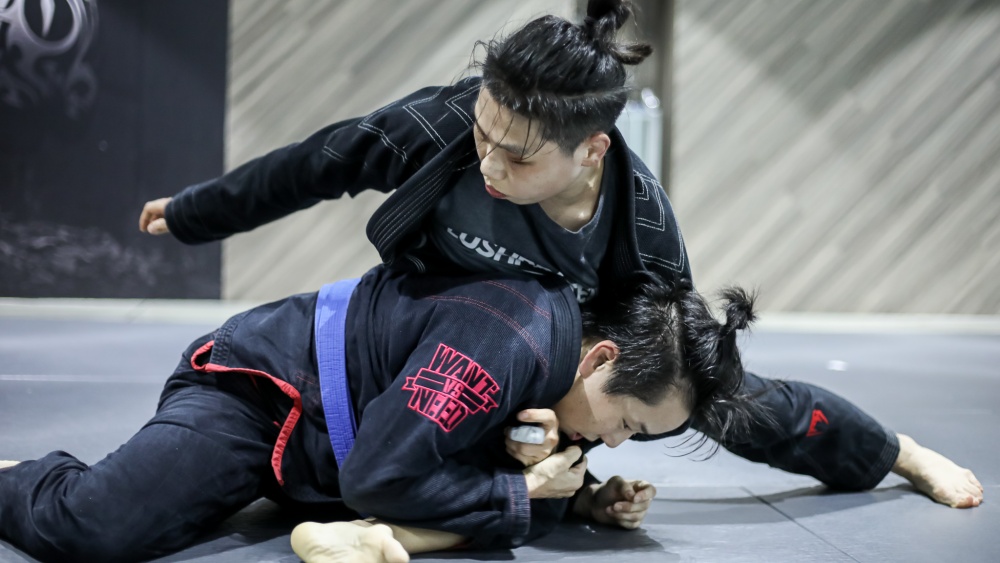In this indoor photograph, two young men of Asian descent are engaged in a martial arts practice, possibly judo or jujitsu, on a gray floor mat. Both wear thick, black martial arts uniforms with t-shirts underneath. The mat extends from the lower edges of the image up to the center, and the background features gray walls with a diagonal pattern and a distant black section in the upper left corner.

The young man on the bottom, with short black hair tied into a top ponytail, wears a uniform with red "Want vs. Need" text on the arm and a blue belt around his waist. He has his left knee bent and is curled over it, with his right leg extended off-screen. The other young man, also with short hair styled into buns or ponytails, lies on top, pinning the first man with one arm beneath his chest. His uniform is adorned with small white chevron stripes, and he also wears a black t-shirt with indistinguishable white print.